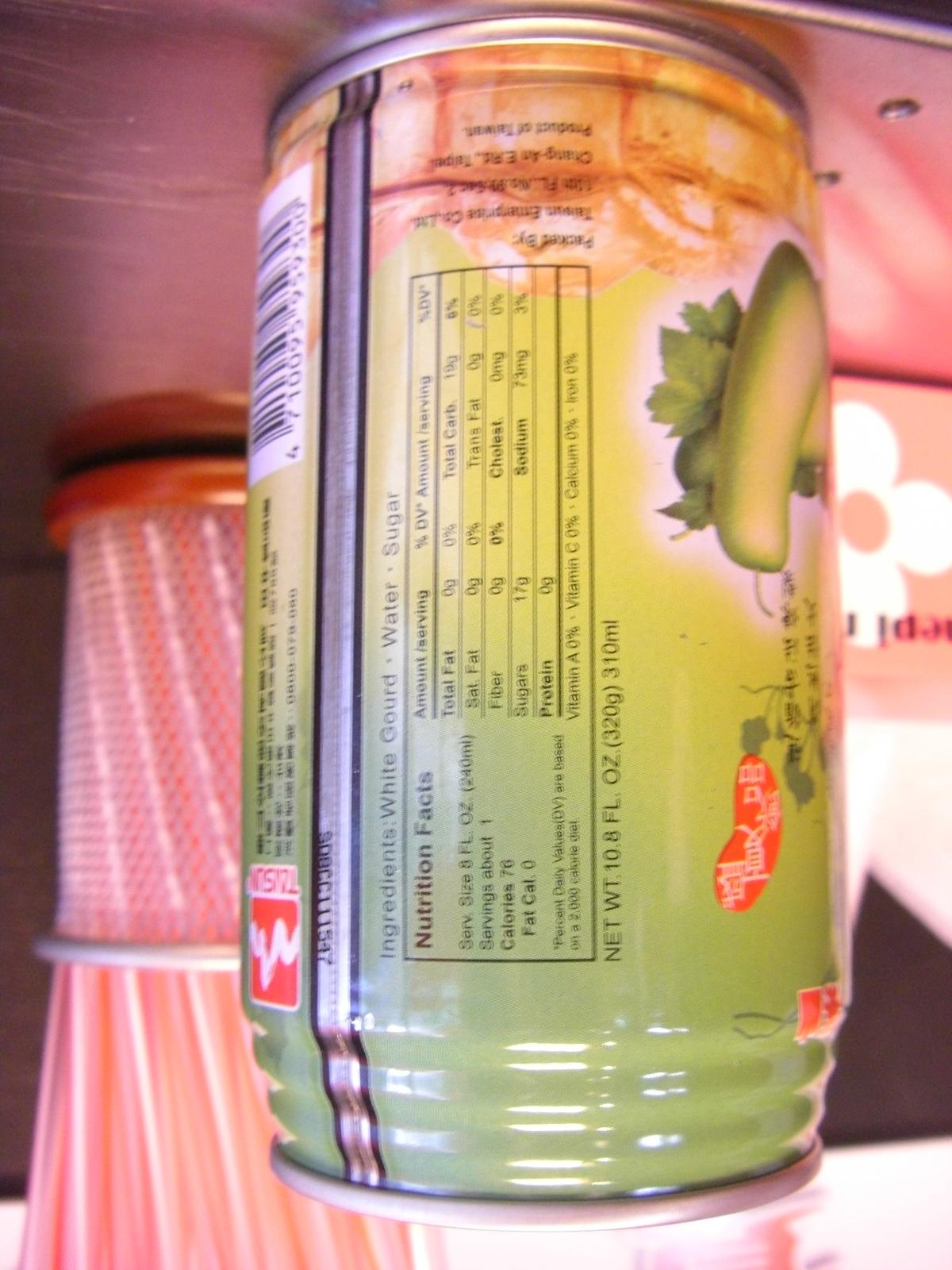An upside-down vertical can featuring a nutrition facts panel on its side dominates the left side of the image. The nutrition facts are oriented towards the top of the screen due to the image being inverted. Adjacent to the misaligned can is a picture of a squash or a long green vegetable with leaves, adding a touch of freshness to the scene. The setting is a rustic wooden table that enhances the natural theme. Positioned behind the can is a small white wire basket with an orange bottom, filled with plastic straws.